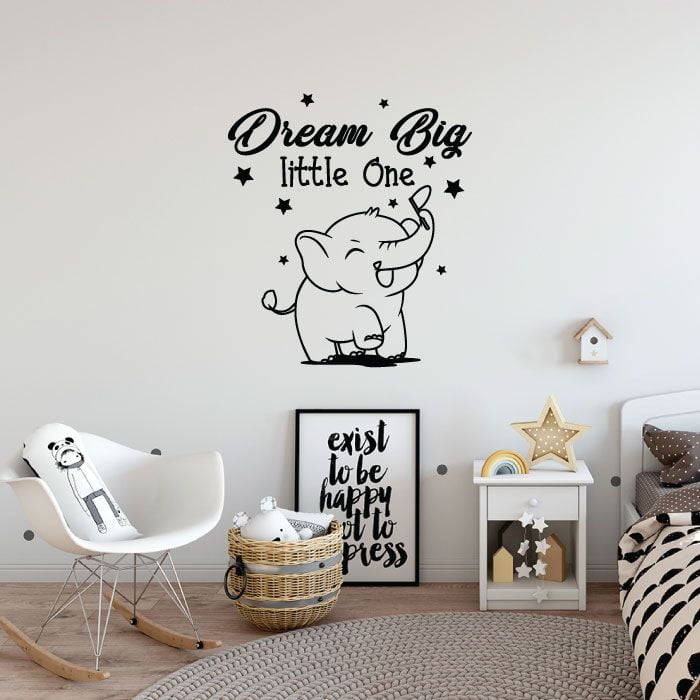The photograph captures the serene and playful ambiance of a child's bedroom with a minimalist yet whimsical decor. Dominating the scene is a pristine white wall adorned with a charming cartoon illustration of a baby elephant, merrily holding up a flag with its trunk and wearing a joyous, closed-eye smile. Above the elephant, the inspirational phrase "Dream Big Little One" is inscribed, surrounded by a sprinkling of black stars. Below the wall art, a framed poster proclaims, "Exist to be happy, not to impress," though the words "not" and "impress" are partially obscured by a wicker basket. This basket houses an adorable white stuffed bear, adding to the room's playful charm.

To the right of this setup, a toddler bed peeks into the frame, featuring an arched white headboard, a monochrome blanket, and brown polka-dotted pillows. Adjacent to the bed, a small nightstand stands with a rainbow figurine, a star light fixture, and a whimsical chain of white stars cascading from its handle. Above this nightstand, a birdhouse with a brown gable and black entry hole is mounted on the wall, enhancing the room's storybook feel.

On the left side of the room, a modern white rocking chair adorned with a monochrome cushion complements the soft beige, wood-like flooring that extends throughout the space. A braided beige rug lies at the center, tying together the room’s cozy, inviting aesthetic. The overall photographic style captures the realism of the scene, highlighting every delightful detail of this thoughtfully arranged space.